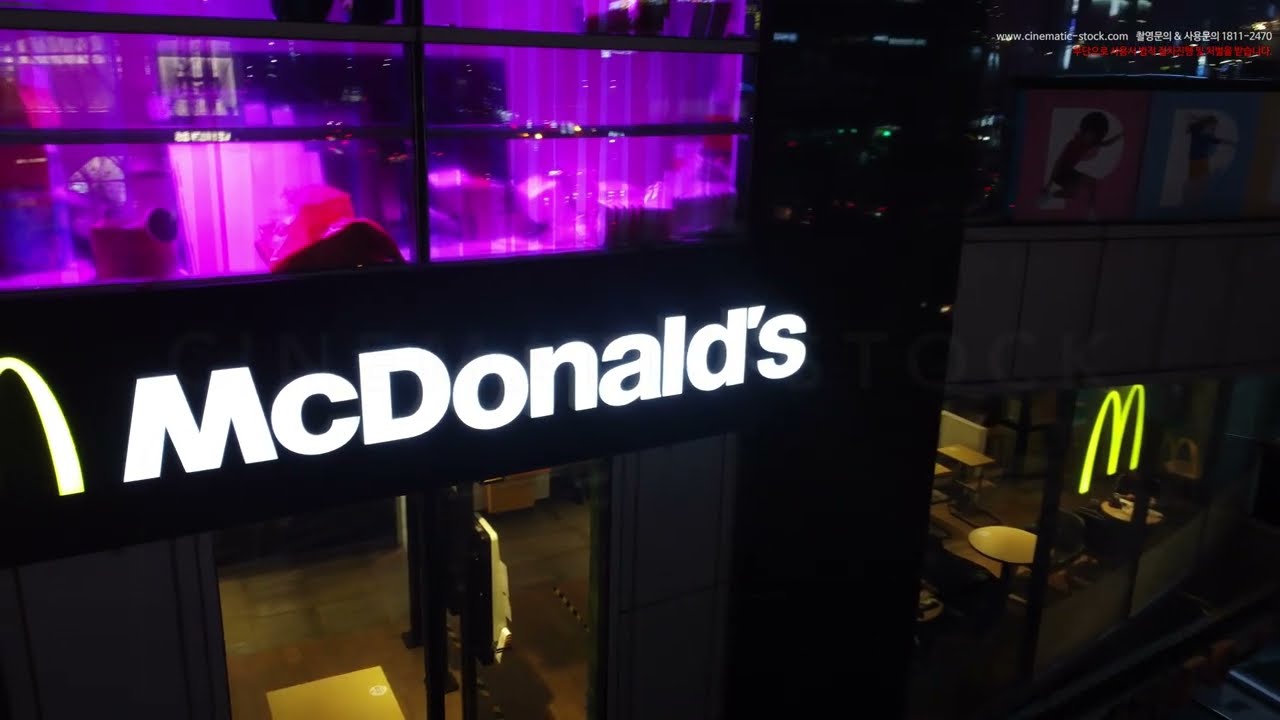This photograph features a modern McDonald's restaurant, likely situated in a large city such as New York, captured during the nighttime which lends a dark atmosphere to the scene. To the left, the McDonald's signage is prominent, though partially obscured with only half of the iconic yellow "M" visible next to the white LED-lit "McDonald's" text. Below this is a set of large glass double doors serving as the main entrance to the restaurant. Above these doors, there's an upper window illuminated with striking pink lights that suggest it might be a bedroom or another private area, casting a fluorescent purple glow outward. On the right side of the image, there's a sign depicting two different women - a black woman encapsulated by pink and a white woman encapsulated by blue, both notably seated on the letter "P". The restaurant's interior can be glimpsed through the windows and appears to have a beige decor, however, the visibility is limited due to the nighttime setting.